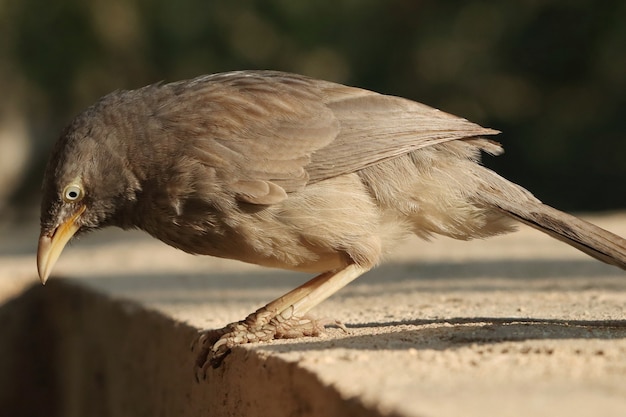In this detailed close-up image, we see a brown bird perched on the edge of a beige, concrete surface. The bird is standing with its toes hanging slightly over the edge, staring intently downwards as if it has spotted something below, perhaps some scattered bird seed or food. The bird features a striking color gradient: its feathers are dark brown on the head and upper breast, transitioning to a lighter brown towards the back and tail. Its beak, resembling the color of wood or a faded orange hue, adds another layer of detail. The bird's eyes are small, black, and beady with a surrounding white, focused downward with great concentration. The background is a mix of muted brown tones and out-of-focus greenery, implying the scene is set in a garden or natural area, enhancing the bird’s earthy colors.